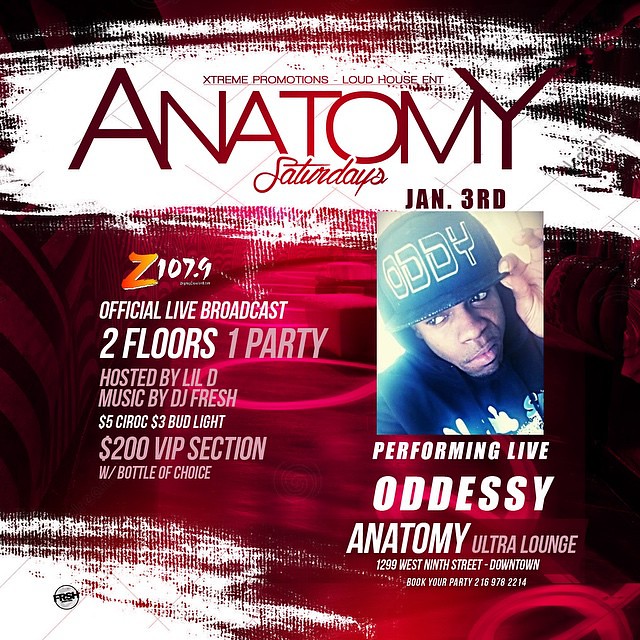This is a color image of a nightclub promotion flyer primarily in a striking red hue with white graphic elements. At the top, white streaks or smears slice through the red background, giving it a dynamic texture. The top text in red reads "Extreme Promotions" and "Loud House Entertainment" in smaller type. Below that, in bold, large fonts, it says "Anatomy," followed by "Saturdays" in a smaller script underneath. The flyer prominently announces "January 3rd" in black text to the right. 

A central feature is a picture of a man wearing an "ODDY" baseball cap, and below his image, it reads "Performing Live Odyssey" at "Anatomy Ultra Lounge." At the flyer’s lower section, detailed event information includes "Z107.9 Official Live Broadcast," "Two Floors, One Party," "$5 Ciroc," "$3 Bud Lights," and "$200 VIP section with a bottle of choice." The overall look is eye-catching, with an abstract red decoration in the middle, creating a vibrant party vibe for a downtown event.